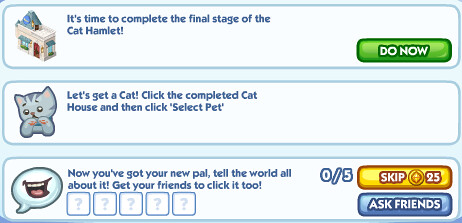The image depicts an animated, game-like interface featuring three horizontally aligned rectangular text boxes, each with a light blue background and a darker blue border. The top text box displays an icon of a building and reads, "It's time to complete the final stage of the Cat Hamlet," with a green "Do Now" button in the corner. The middle text box shows an animated gray cat with its paws up, instructing players to "Let's get a cat. Click the completed cat house, and then click Select Pet.” The bottom text box features a chat bubble icon with an open mouth, advising, "Now you've got your new pal. Tell the world all about it. Get your friends to click it too." Below this message, there are five empty boxes marked with question marks and a counter reading "0/5." To the bottom right, a yellow "Skip" button costing 25 gold coins is visible, along with a blue "Ask Friends" button. The image is accented with various shades of blue, yellow, green, and brown.